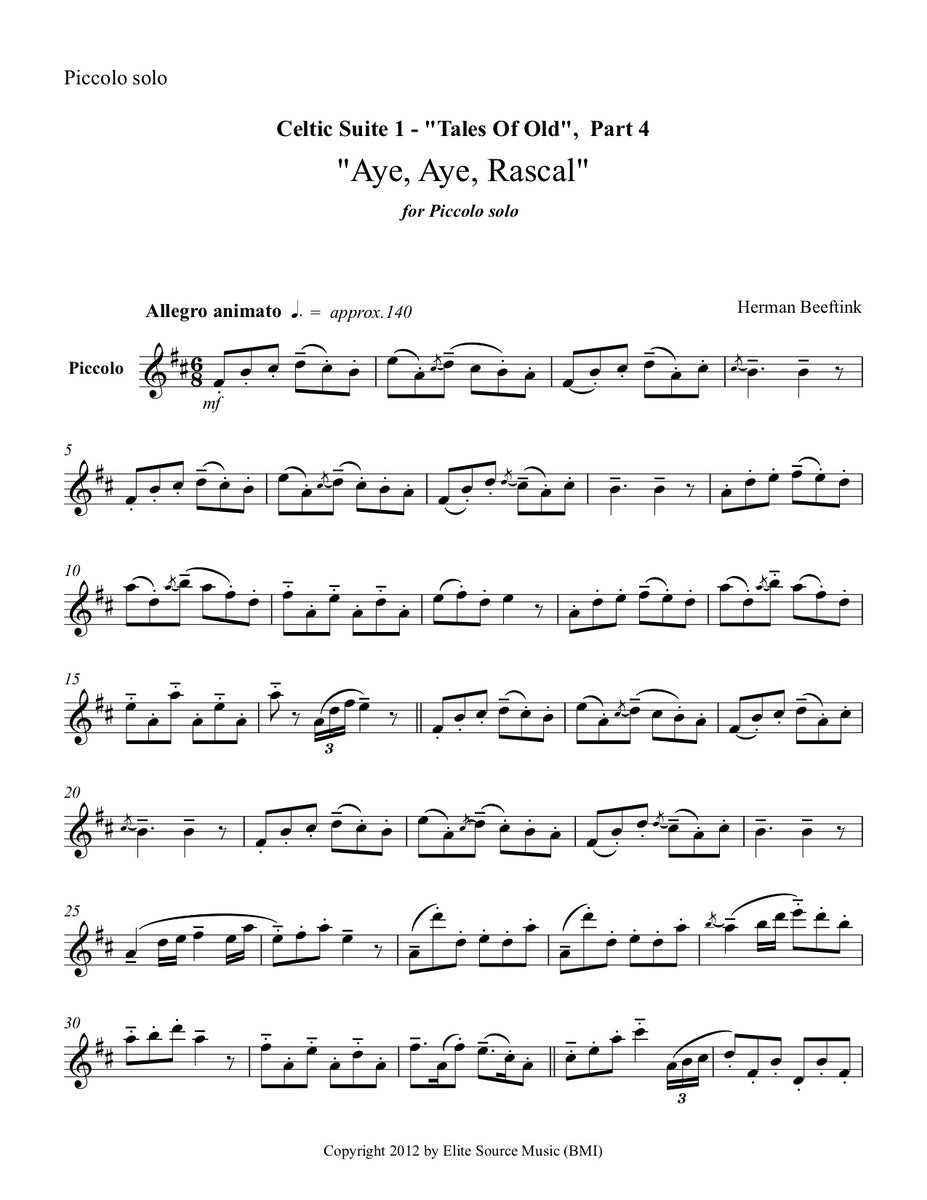The black-and-white image depicts a vertically rectangular sheet of music without a border, set against a white background. In the upper left-hand corner, it reads "Piccolo Solo." Centered at the top, three lines of text state "Celtic Suite I – 'Tales of Old,' Part IV: 'I, I, Rascal,'" followed by "for Piccolo Solo." To the right, the name "Herman Beef Tank" appears above the staff. Below this, "Allegro animato ≈ 140" indicates the tempo and style. The sheet includes musical notation spread over seven lines, each marked at the left with numbers in increments of five. The bottom center of the page notes "Copyright 2012 by E-Line Source Music, BMI." This sheet music is intended to be played on the piccolo, as indicated by the instrument reference at various points across the page.